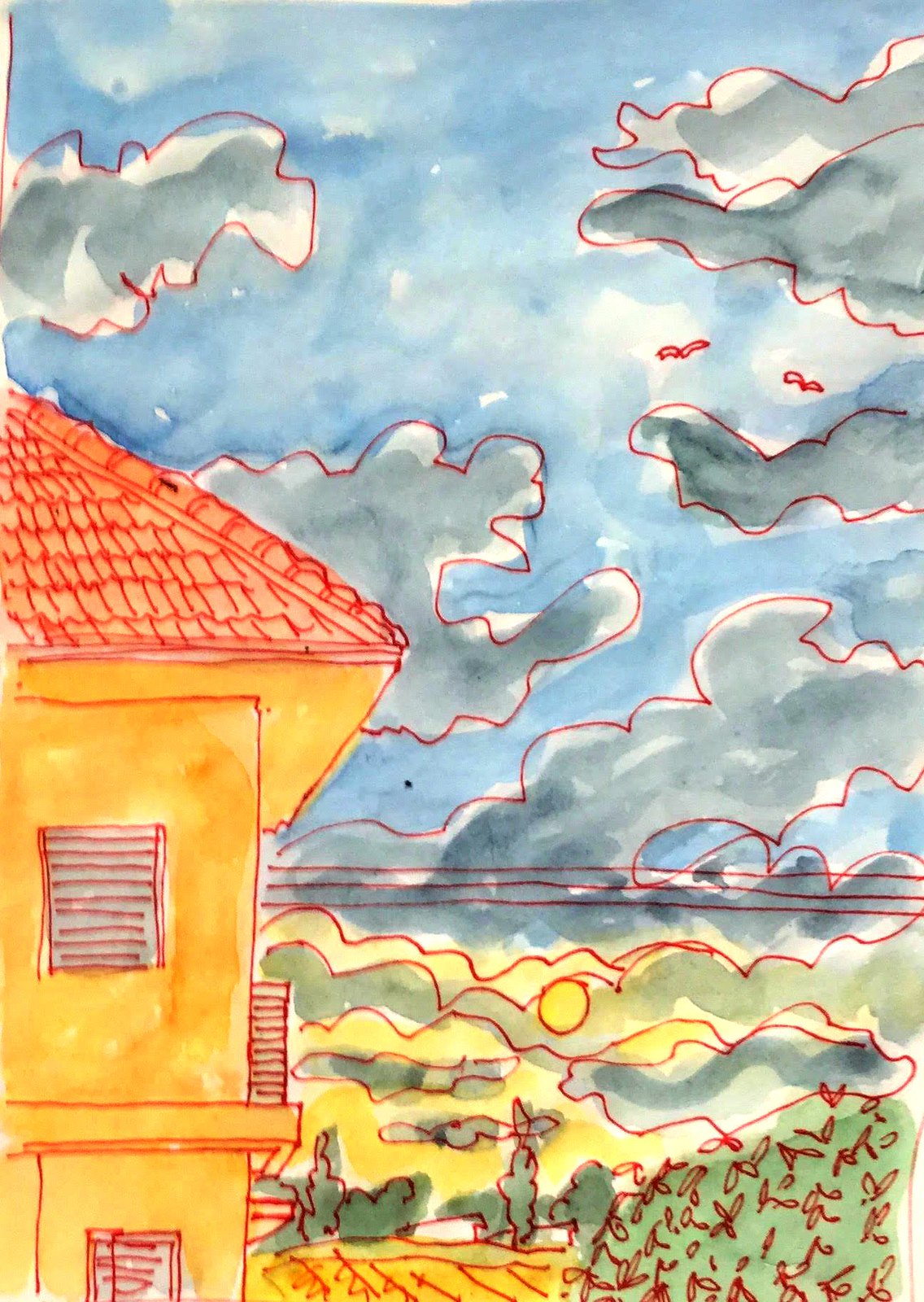The image appears to be a child's watercolor painting on a wide piece of paper. The artwork features a yellow two-story house located in the lower left-hand corner, with visible shingles on the roof and horizontal lines representing windows complete with shades. The sky is painted blue with gray clouds that have been outlined in red ink. Additionally, there are rudimentary birds, depicted as simple swoops, flying in the sky. A green bush can be seen near the house, also outlined in red. The overall simplicity and rough style of the details, such as the red ink outlines around various elements, suggest the painting was done by a child.